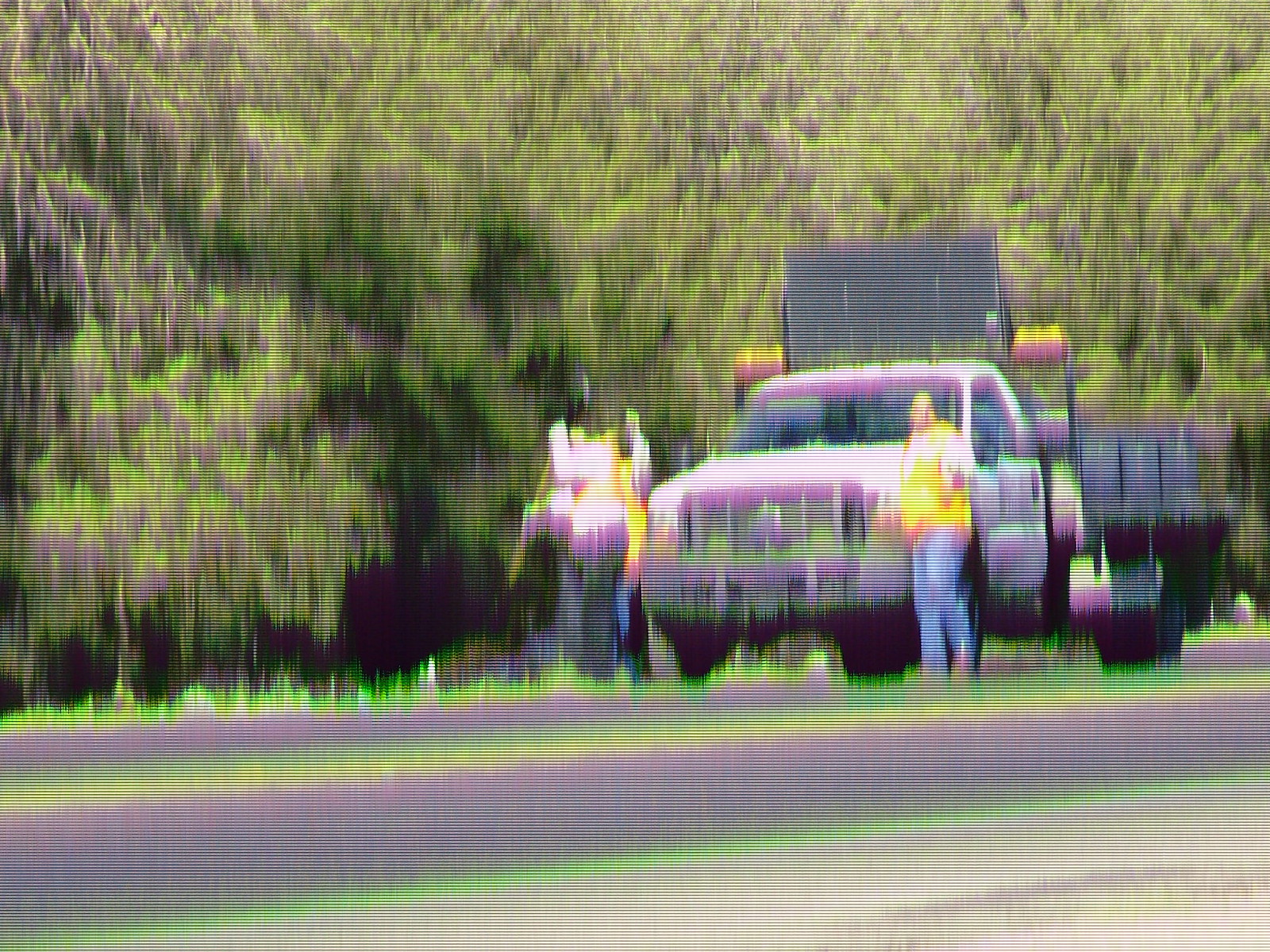This very blurry photograph, which appears to be taken from a car window or possibly a screen, depicts a scene on the side of a two-lane highway with a yellow stripe down the middle. On the opposite side of the road, a white road service truck is parked, along with a black dump truck. Surrounding the trucks are at least three workers, distinguished by their attire. The worker nearest the camera, standing by the dump truck, is dressed in a yellow vest, white shirt, blue jeans, and boots. Another worker on the opposite side of the dump truck appears to be holding a tool, likely a shovel, and is also wearing a distinct vest and white shirt, although his vest's color varies in the descriptions. Behind him, there is a third worker in a yellow vest. The image erroneously displays horizontal lines as if taken from a screen or printed with low ink, further blurring the details. The background features a tree-covered hillside, adding a natural backdrop to the work scene.